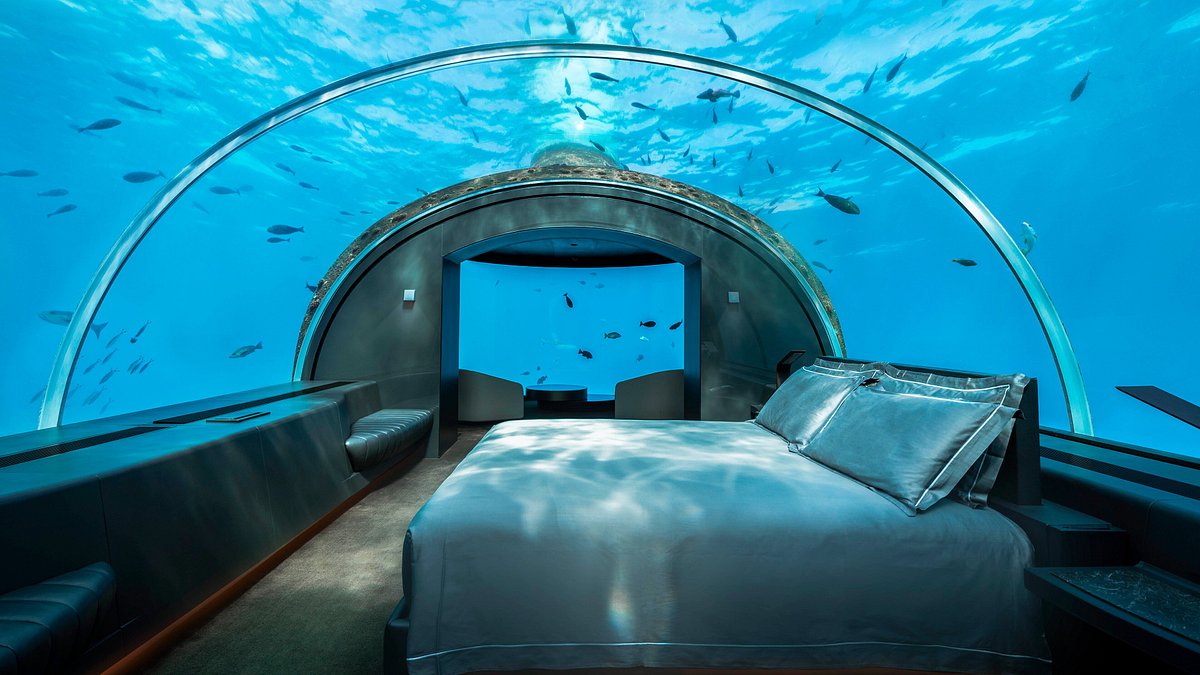The image showcases an underwater hotel room encased in a clear glass dome, providing an unobstructed view of the surrounding ocean. The room, resembling a long cylindrical tube, features a simplistic design with a large queen-size bed placed toward the right side of the dome, oriented so that the feet of the bed face left. The bed is dressed in dark gray covers and pillows, with two pillows propped up against the headboard. Beside the bed is a counter shelf, perhaps for small personal items.

Beyond the room's transparent walls, you can observe a multitude of small, elongated fish, including what appears to be sea bass, swimming in the pristine blue water. The fish, which seem to range in color from black to more varied hues, are visible on all sides of the dome. The ceiling and side walls of the hotel room arch gracefully overhead, and through the glass, you can see the surface of the water with occasional waves and whitecaps. In the background, the sunlight faintly penetrates the water, illuminating the scene with a gentle glow.

The simplicity of the room's interior, devoid of conventional artwork, emphasizes the natural beauty outside, making the moving sea life the focal point of this unique underwater experience. There is also another section at the end of the room, seemingly encased in concrete with a see-through glass end, allowing for additional views of the underwater scenery and more fish swimming peacefully by.